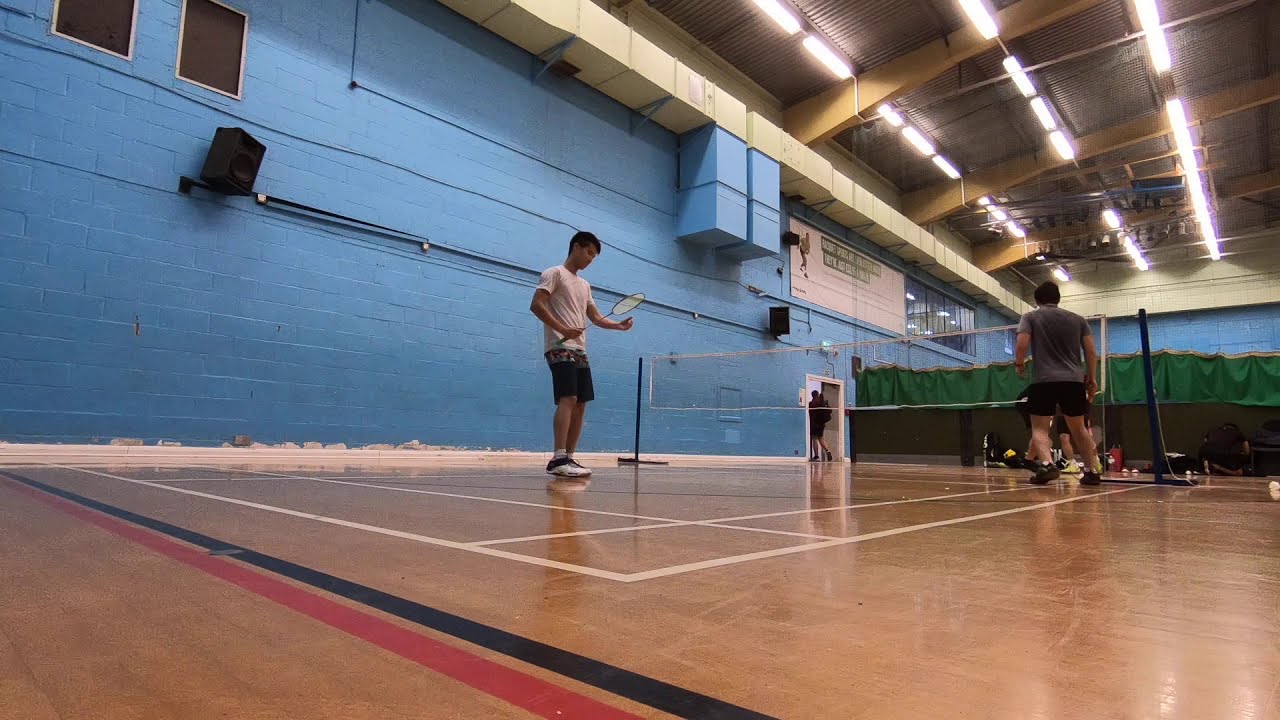The image depicts the interior of a gymnasium with a high ceiling featuring exposed yellow metal rafters and fluorescent lighting. The walls are painted a sky blue, and there are visible air conditioning ducts overhead. The wooden floor of the gymnasium is slightly scuffed and marked with various colored stripes, including red, black, and white lines that designate a badminton court. 

In the foreground, a young man wearing a white t-shirt and black shorts holds a badminton racket, poised to serve. Another player in a gray shirt and black shorts stands closer to the net, which has a white mesh and dark posts. Their positioning partly obscures the other players on the opposite side of the court. The vantage point offers an oblique angle from one side of the net, revealing a brightly varnished tan floor and a doorway in the background through which a person is walking. Overall, the gym's institutional design and cinder block construction are evident, creating a functional yet straightforward sports environment.